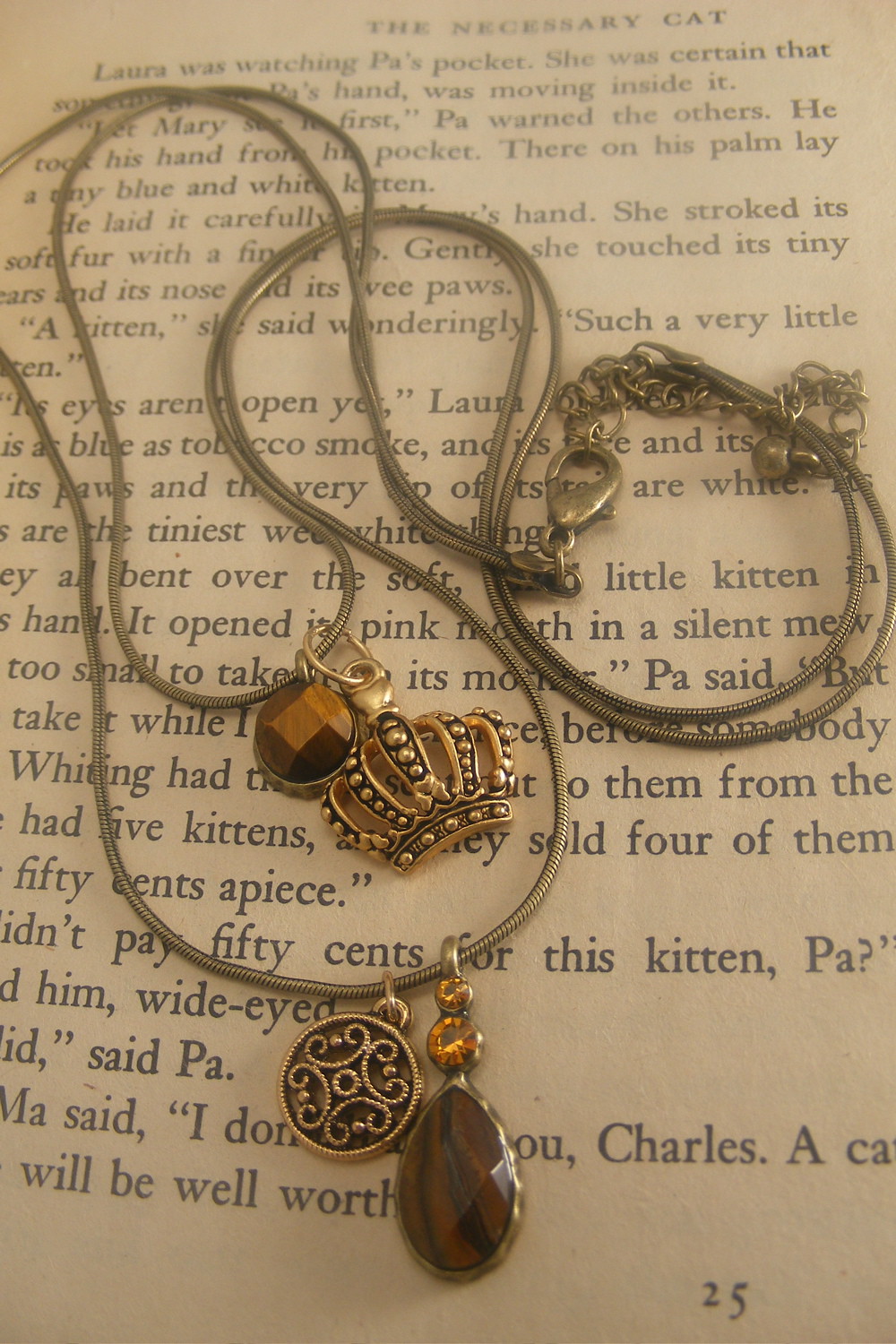The image depicts a photograph of a necklace placed on an open page of a book. The necklace, which rests prominently at the center of the beige-pink page, features a black or possibly metallic cord with a lobster claw closure. Adorning the necklace are four distinct charms: a gold crown, a circular pendant that appears to be wooden or a faux gemstone in brown, a shield-shaped charm in gold, and a darker brown faux gemstone shaped like a teardrop with two smaller circles above it. The page, numbered 25, includes black serif-style text from a story titled "The Necessary Cat," with a legible excerpt about a character named Pa holding a tiny blue and white kitten in his palm. The overall setting seems to be indoors, capturing a moment where the necklace was delicately placed atop a book, enhancing the intricate details of both the jewelry and the text.